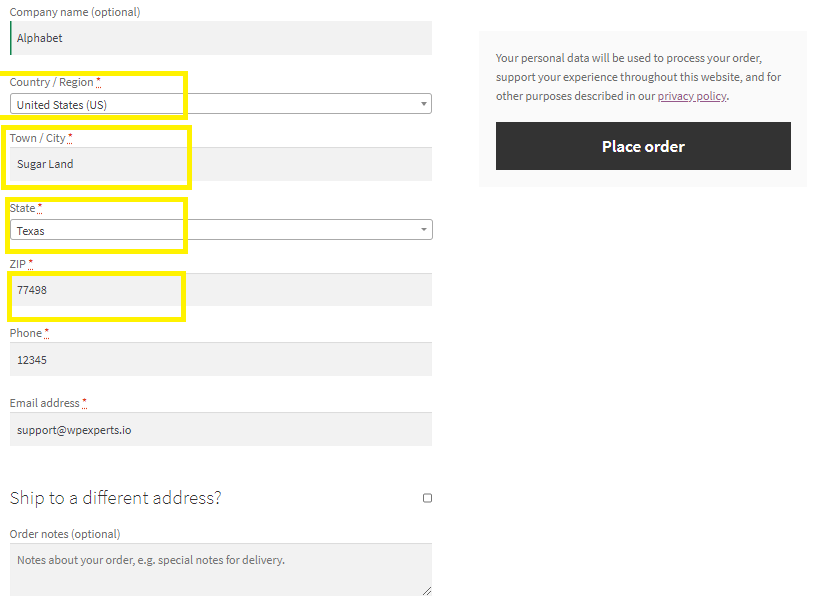In the image, the company's name appears on the upper left-hand side, written in a gray font. The name is enclosed in parentheses, and an optional label follows it, also in gray. Below this, a gray bar extends from left to right, displaying the word "Alphabet" in uppercase letters. There's a thin greenish line on the left edge of this bar, which is part of the bar's design. 

Underneath the bar, there is a drop-down arrow beside a section labeled "Country/Region" with a red asterisk indicating it is a required field. The selection box next to this label displays "United States" followed by "(US)" to denote the chosen country. 

Moving downward, another box is labeled "Town/City," also marked with a red asterisk. "Sugarland" is typed in black text inside this box. Below this is a section for the "State," which features a drop-down arrow where "Texas" has been selected. Lastly, the "Zip" section contains the postal code "77498" that has been entered in numeric form.